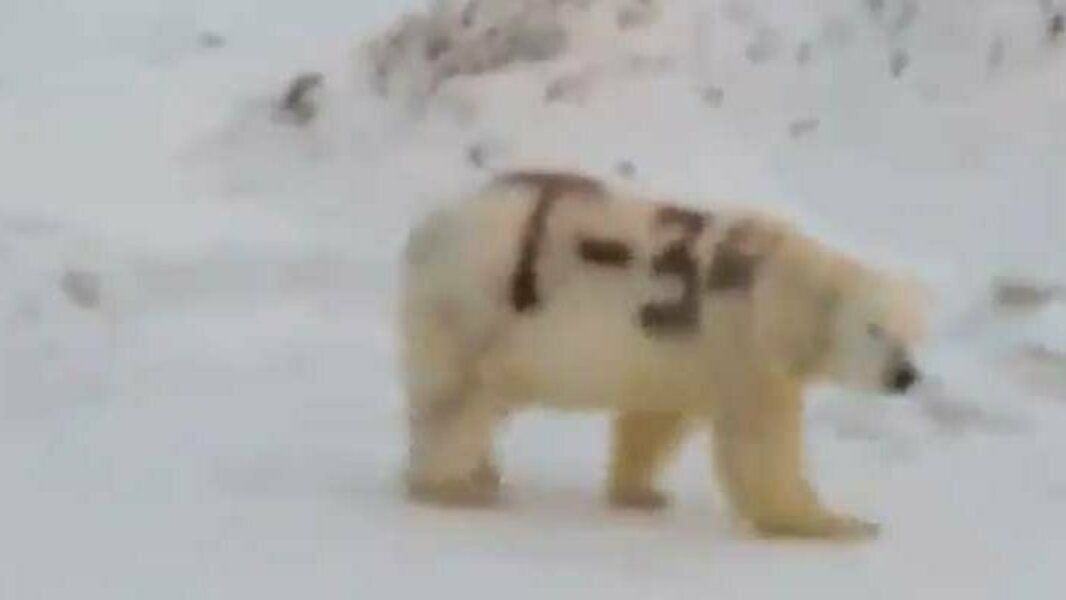A grainy and blurry photograph captures a polar bear walking towards the right. The image makes it challenging to discern fine details. The bear’s right paw is extended farther than its left, and only one of its hind legs is visible. Disturbingly, the bear has been marked with black spray paint across its back, which reads "T/3". There is an additional, unidentifiable mark. The bear’s nose is black, and while its face and sides are predominantly white, there are light brown tones around its legs and neck. In the background, gray rocks suggest the side of a hill, partially covered in snow.